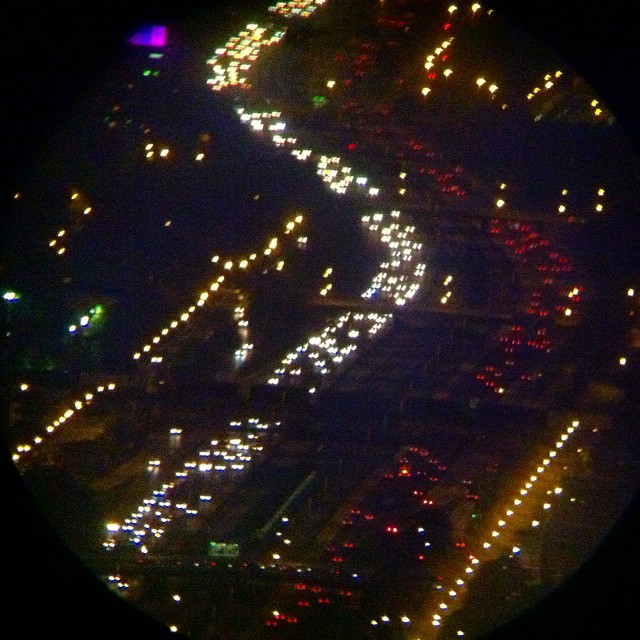This photograph, taken at night from a high vantage point—possibly an airplane or a tall skyscraper—captures a bustling city freeway several hundred feet below. The image, slightly blurred due to the low light conditions, showcases a large, S-shaped highway with six lanes divided into two distinct directions of traffic. On the left side of the image, the stream of white headlights from countless cars indicates traffic heading in one direction, while on the right side, a sea of red taillights marks the flow of vehicles in the opposite direction. Additional points of interest include dimly lit bridges and scattered lights, possibly from street lamps and vehicle lights, as well as a large green highway sign that provides location and distance information. The top left corner features a purple and violet triangular object, adding a unique element to the scene. The congested traffic, likely from rush hour or an event, highlights the city's vibrant nocturnal activity.